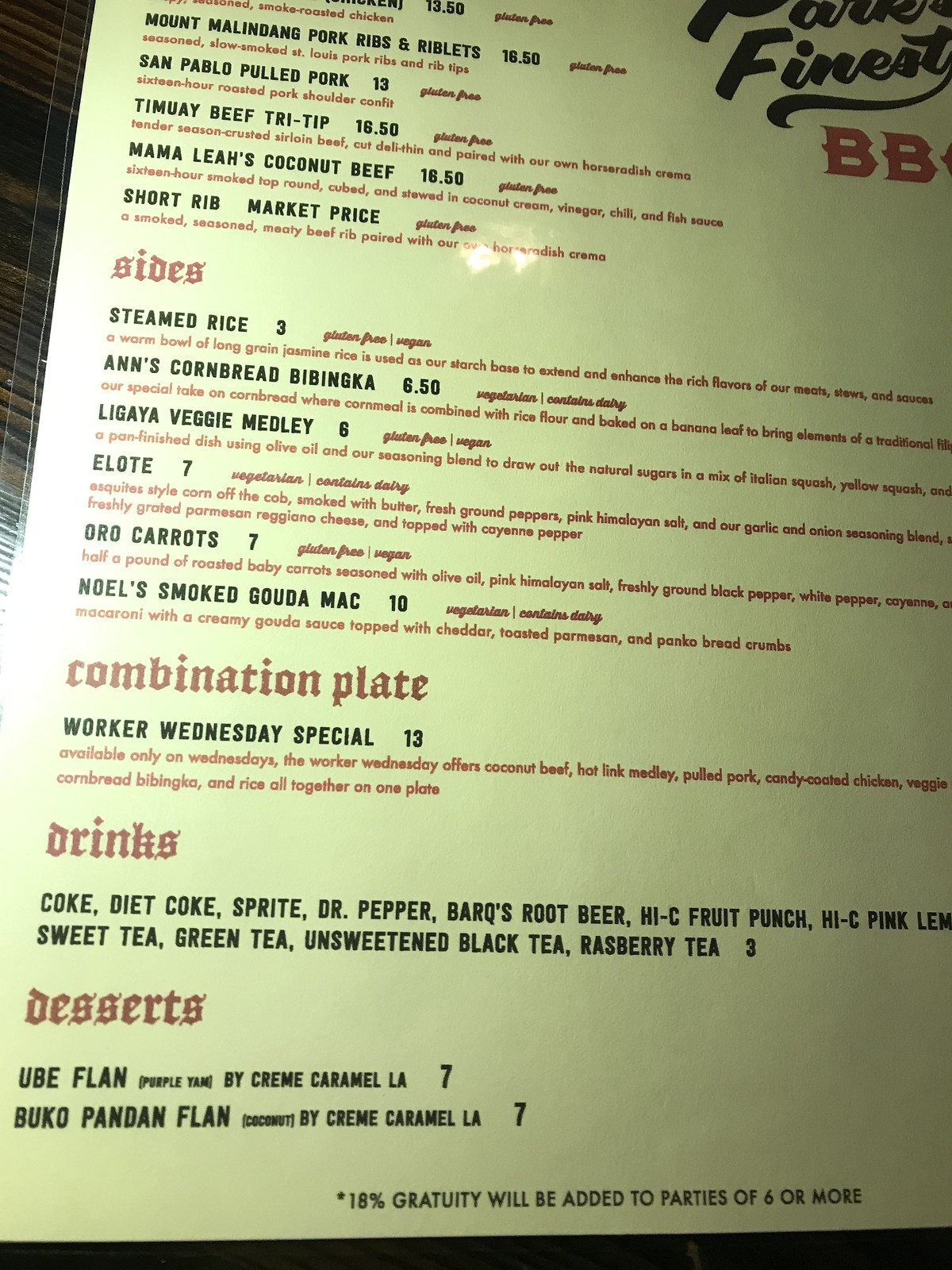This detailed photograph showcases a laminated menu of a barbecue restaurant, likely named "Park's Finest Barbecue," although the restaurant's full name is partially cut off in the top right corner. The menu lies on a rustic wooden table. The visible portions of the menu include a variety of mouthwatering entrees and sides, along with combination plates, drinks, and desserts.

The entree section, visible in the top left though partially cut off, features items such as:
- Mount Malindang Pork Ribs and Riblets: $16.50
- San Pablo Pulled Pork: $13.00
- Timoy Beef Tri-Tip: $16.50
- Mama Lea's Coconut Beef: $16.50
- Short Rib: Market Price
  
Accompanying the entrees, an array of delectable sides is also listed:
- Steamed Rice: $3.00
- Cornbreads, Babinka: $6.50
- Ligaya Veggie Medley: $6.00
- Elote: $7.00
- Oro Carrots: $7.00
- Knoll's Smoked Gouda Mac: $10.00

The next section of the menu highlights a notable "Combination Plate" under a special offer termed "Worker Wednesday Special" priced at $13.00. This plate includes a mix of Coconut Beef, Hot Link Medley, Pulled Pork, Candy Coated Chicken, Veggie, Cornbread, Babinka, and Rice all together.

A selection of beverages follows, offering a variety of choices:
- Coke
- Diet Coke
- Sprite
- Dr. Pepper
- Barq's Root Beer
- Hi-C Fruit Punch
- Hi-C Pink Lemonade
- Sweet Tea
- Green Tea
- Unsweetened Black Tea
- Raspberry Tea

For dessert enthusiasts, the menu features:
- Ube Flan: $7.00
- Buko Pandan Flan: $7.00

Finally, a note at the bottom of the menu indicates that an 18% gratuity will be added to parties of six or more. The enticing offerings and careful detail in the menu layout tease a delightful dining experience at this barbecue haven.